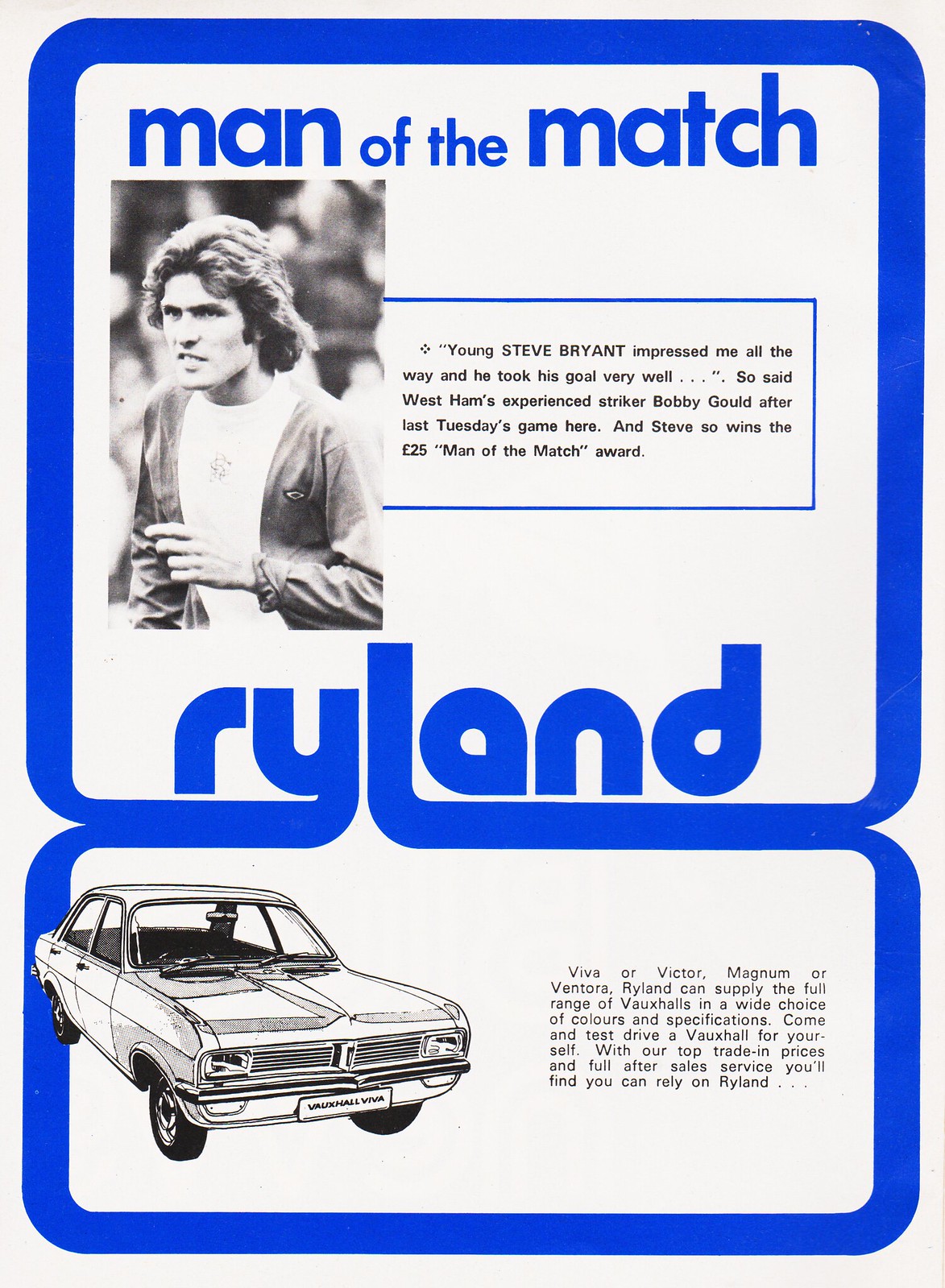The poster is an old, paper-sized scan with a white background and a royal blue outline. At the top, in royal blue text, it reads "Man of the Match." Below this title, the name "Ryland" is prominently displayed in large, bold letters. The poster features two main images: a black-and-white photograph of a young white man with just-above-shoulder-length hair, wearing a white shirt with a grayish cardigan, and a sketch of a car at the bottom. 

To the right of the man's photo, enclosed in a blue-outlined box, there is a paragraph that reads: "Young Steve Bryant impressed me all the way, and he took his goal very well," said West Ham's experienced striker Bobby Gould after last Tuesday's game. "And Steve so wins the £25 Man of the Match award."

Beneath the man's information, the text reads: "Ryland. Viva or Victor, Magnum or Ventura, Ryland can supply the full range of voxels in a wide choice of colors and specifications. Come and test drive a voxel for yourself. With our top trade-in prices and full after-sales service, you'll find you can rely on Ryland." The car sketch is positioned to the left of this text, completing the advertisement.